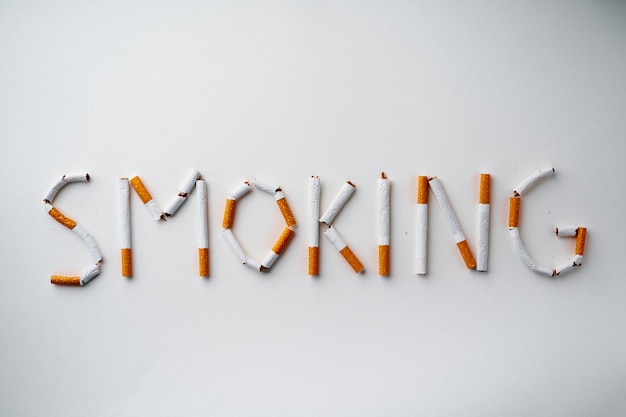This horizontal rectangular image features the word "smoking" spelled out intricately with broken cigarettes against a plain white to gray gradient background. Each letter of the word is crafted using multiple cigarettes: the "S" is formed by creatively bending and segmenting the cigarettes, placing the orange filters at the bottom and curving the white tobacco parts to shape the letter. The straight letters like "I" and "N" are composed of cigarettes laid end-to-end, while others like "O" and "G" utilize extra pieces of the cigarettes to achieve the necessary curves and shapes. The backdrop subtly transitions from darker tones on the top and bottom edges to a lighter center, highlighting the detailed construction of the cigarette-formed letters, reinforcing a possible message about the destructiveness of smoking.